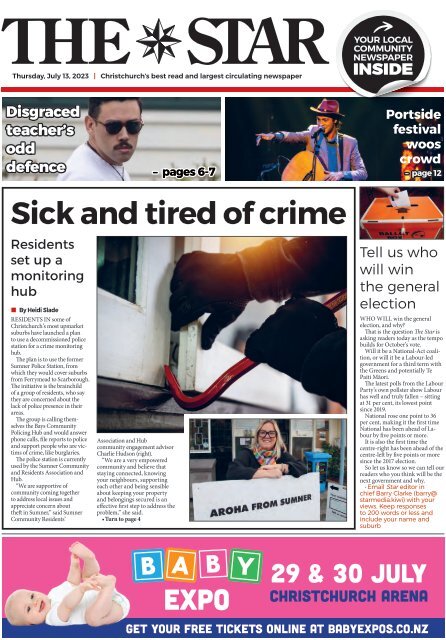This image is the front page of the "Star," your local community newspaper in Christchurch, New Zealand, dated Thursday, July 13th, 2023. 

Headlining the edition, there is a prominent article titled “Sick and Tired of Crime: Residents Set Up a Monitoring Hub,” accompanied by an impactful photograph. The image depicts an individual attempting to break into a property, using a jimmy to force open a window, illustrating the urgency and gravity of the crime issue addressed in the article.

At the bottom of the page, a vivid pink banner advertises the upcoming Baby Expo, scheduled for the 29th and 30th of July at the Christchurch Arena. The advertisement features a picture of a chubby, joyful baby lying on its back and happily playing with its toes, emphasizing the family-friendly nature of the event. Those interested are encouraged to get their free tickets online at babyexpos.co.nz. 

The "Star" prides itself on being Christchurch's best-read newspaper with the largest circulation, providing vital and engaging community news.